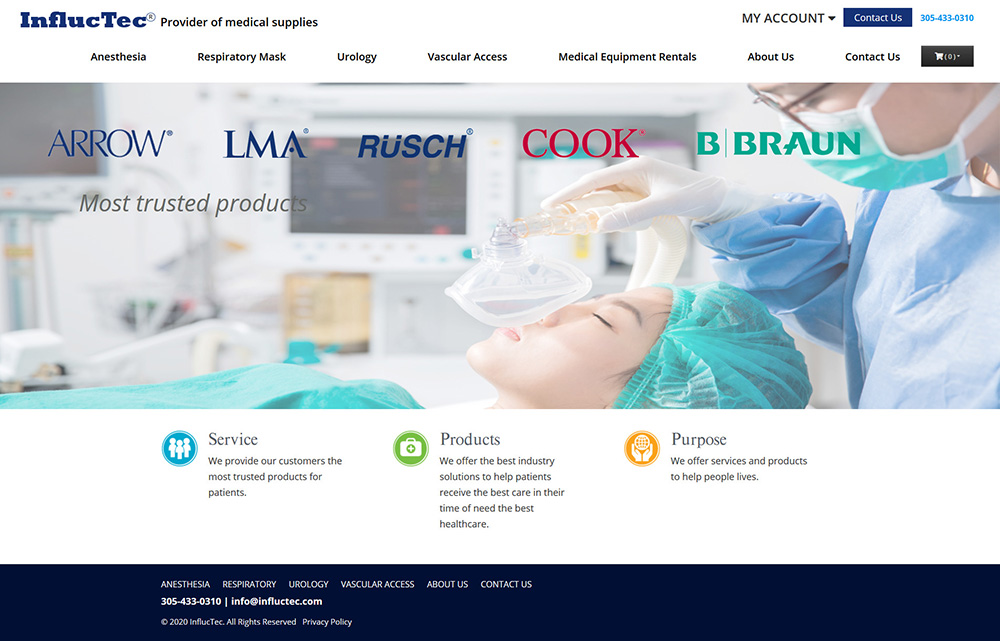The website for Influctech—a trademarked provider of medical supplies—is prominently displayed. The brand name is styled as "Influctech," with a capital "I" followed by "N-F-L-U-C" and a capital "T-E-C" ending in a circled "R" to indicate its registered trademark status. In the upper right corner of the webpage, there are options for "My Account" and "Contact Us," alongside a contact number: 385-433-0310.

The navigation menu spans the top of the site, offering categories such as Anesthesia, Respiratory Mask, Urology, Vascular Access, Medical Equipment Rentals, About Us, and Contact Us. Central to the webpage is an image depicting a patient, who appears to be an Asian woman dressed in green scrubs and a green hairnet. An anesthesiologist is attentively administering anesthesia with a clear mask over her face. The image is captioned with "Most Trusted Product" and lists notable brands: Arrow, LMA, RUSCH, Cooke, and B. Braun.

Below the image are three buttons detailing Influctech's offerings:
1. "Service" – Highlighting their commitment to providing customers with the most trusted products for patients.
2. "Products" – A green button describing the company's industry solutions aimed at ensuring patients receive top-tier health care during their times of need.
3. "Purpose" – A yellow-orange button emphasizing their mission to offer services and products that improve people's lives.

At the very bottom of the page, a banner reiterates the main categories: Anesthesia, Respiratory, Urology, Vascular Access, About Us, and Contact. The footer includes the contact number (385-433-0310), an email address (info@influtech.com), and a copyright message.